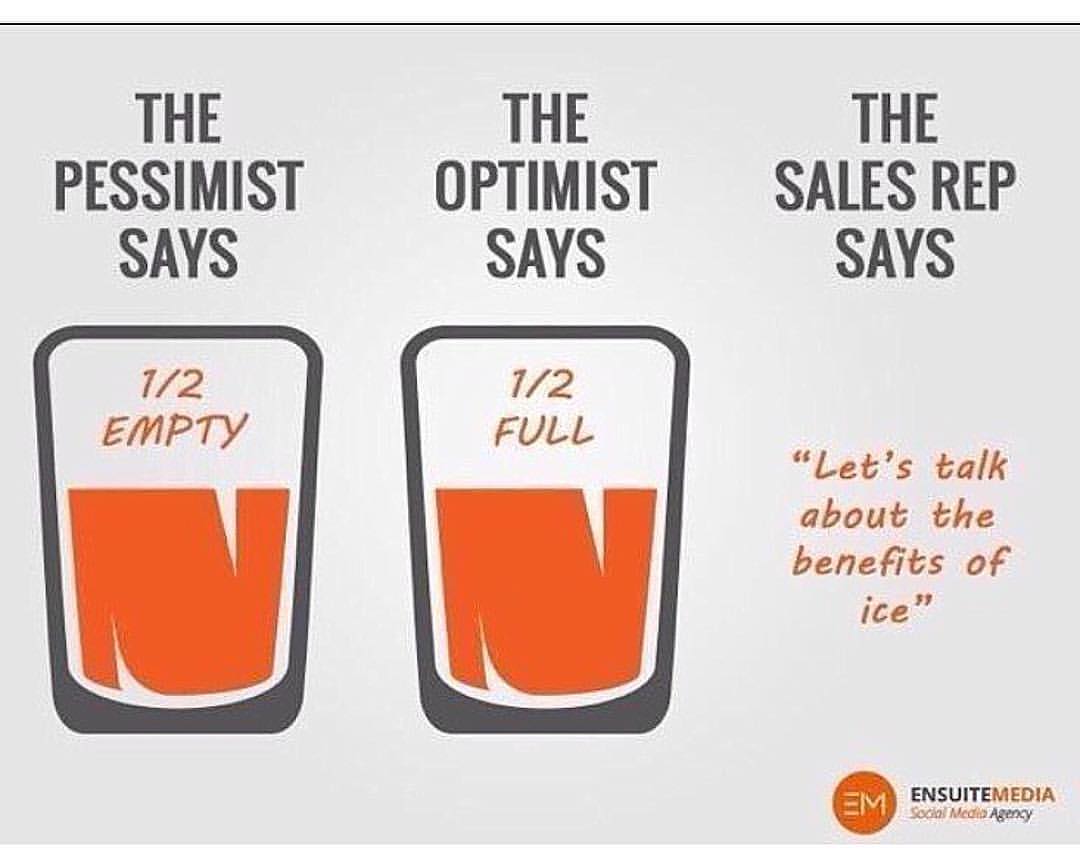The marketing poster features a light gray background and is divided into three equal vertical sections. The left section shows black text at the top reading "The Pessimist Says," with an image of a glass containing orange liquid. The glass, outlined in black, has the text "1/2 Empty" in orange inside it. The middle section mirrors the first, but the black text at the top reads "The Optimist Says." The glass in this section is also half-filled with an orange liquid but has the text "1/2 Full" in orange inside it. The right section's black text reads "The Sales Rep Says," followed by "Let's talk about the benefits of ice" in orange font. There's also a note in the bottom right corner mentioning "EM and Sweet Media, social media agency," in smaller text. The overall design of the poster is somewhat blurry or grainy around the edges of the images and text, giving it an artistic, stylized look.